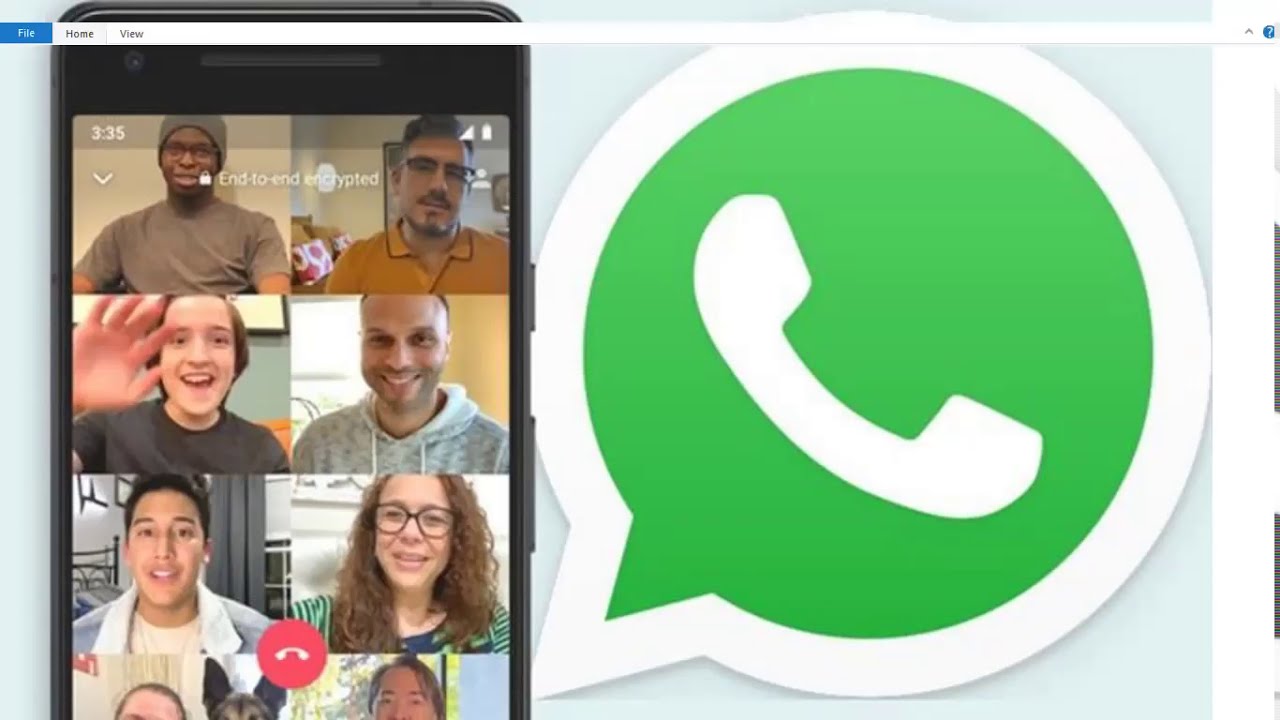The image displays a cellphone screen set against a blue background, showing a video chat interface with eight participants. The upper left corner of the screen indicates "3:35" and the phrase "end-to-end encrypted" is visible, suggesting a secure communication app. The participants are arranged clockwise starting from the top left: 

1. An African-American man with a gray shirt and cap.
2. A man in a mustard-colored collared shirt wearing glasses.
3. A person with brown hair, waving enthusiastically, gender unclear.
4. A man in a gray hoodie, smiling.
5. A middle-aged woman with lightly curled brown hair and glasses.
6. Another man with dark brown hair wearing a light gray jacket.
7. A man with dark hair, wearing a green and lighter green striped shirt.
8. A child with brown hair in a blue coat, waving.

The lower part of the cellphone screen displays a red circle with a white phone receiver, indicating an option to end the call. Adjacent to the cellphone on the right side of the image, there's a large green speech bubble with a white telephone icon inside. At the top of the screen, menu options "File," "Home," and "View" are visible, suggesting this is a screenshot from a digital communication application, where people are connecting from their homes.